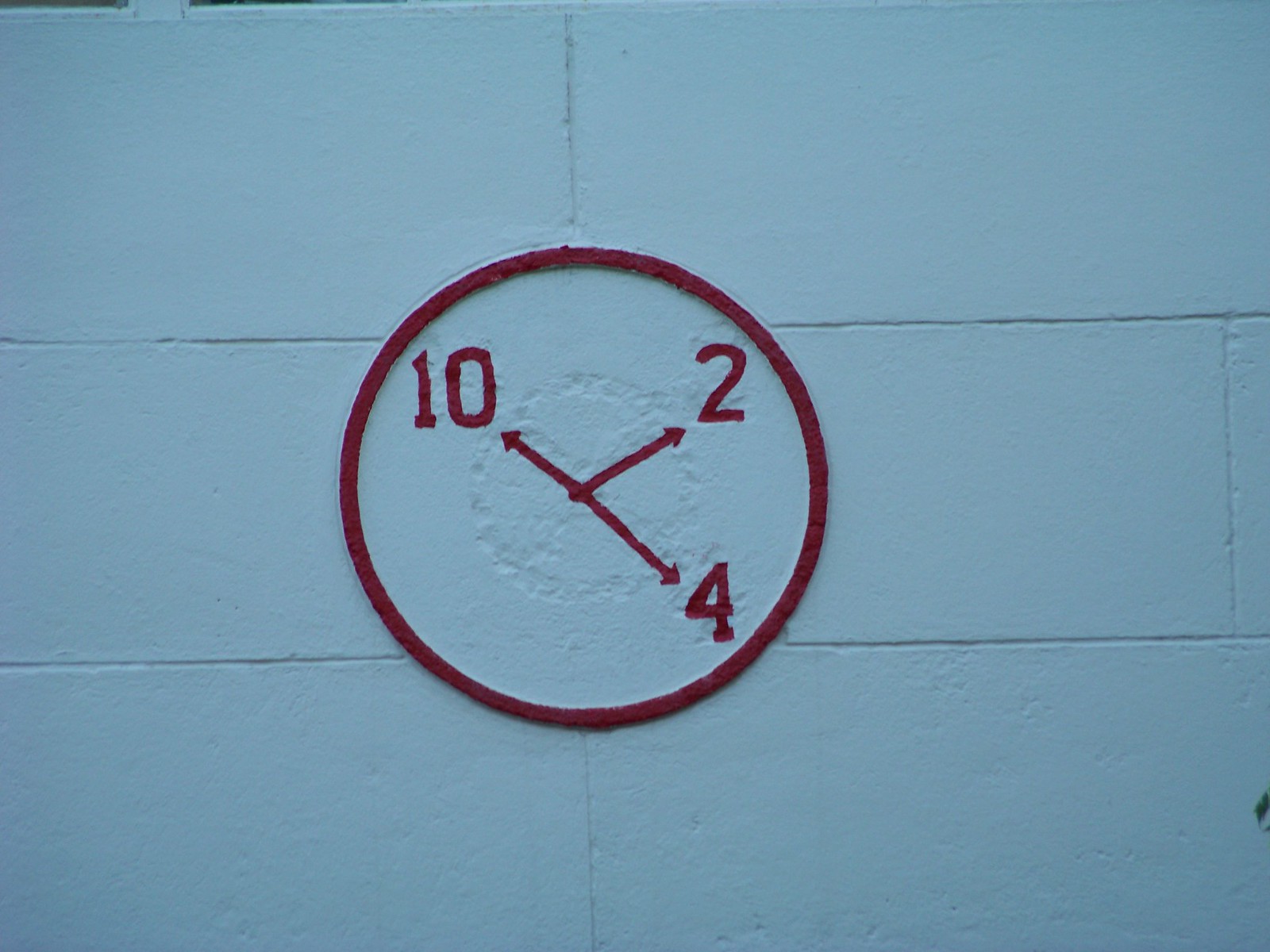This photograph showcases a clock illustration painted on a white-painted concrete block wall, where the individual blocks and their intersections are clearly visible. The wall's original gray-green color subtly peeks through the white paint. At the center of the image is a large red circle, representing the face of a clock. Inside the circle, the numbers 10, 2, and 4 are marked at their appropriate positions on the clock face. Three red lines, resembling clock hands, originate from the center of the circle and point to each of these numbers. The clock face appears slightly worn or scratched, adding a sense of age or texture to the illustration.